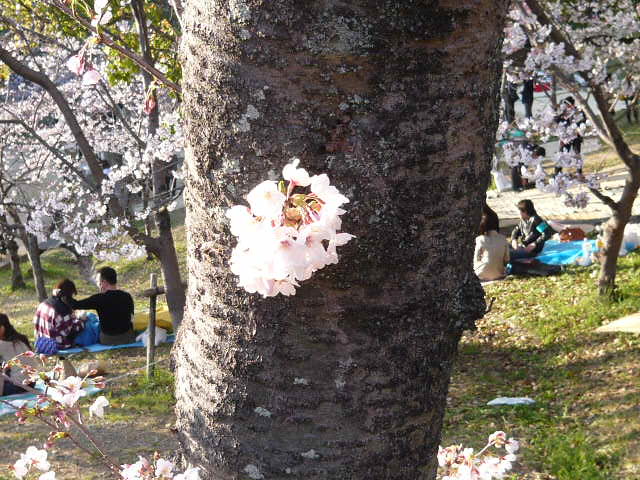In this outdoor image, the central focus is on a large tree trunk that extends vertically through the middle of the photo, disappearing beyond both the top and bottom edges. The trunk features a white cherry blossom flower, possibly stuck to it. Surrounding this tree, the scene is vibrant with springtime flora and activities. To the left of the trunk, the ground is sparsely covered with grass and gravel, leading up to another tree adorned with white flowering buds. Near this location, a man in black is seated on a blue blanket with his arm around a woman in a checkered white and purple shirt. Further to the left, there is an additional person partially out of frame. 

On the right side of the image, another tree is visible, also bearing cherry blossoms. Near this area, two women are seated and conversing, one in a beige dress and the other in a black jacket. The foreground at the bottom of the image reveals more branches and pink flowers, enhancing the floral theme. Moving upwards, the background shows more people—some sitting, others standing—amidst a landscape of lush grass and various blossoming trees, possibly within a park or a graveyard setting.